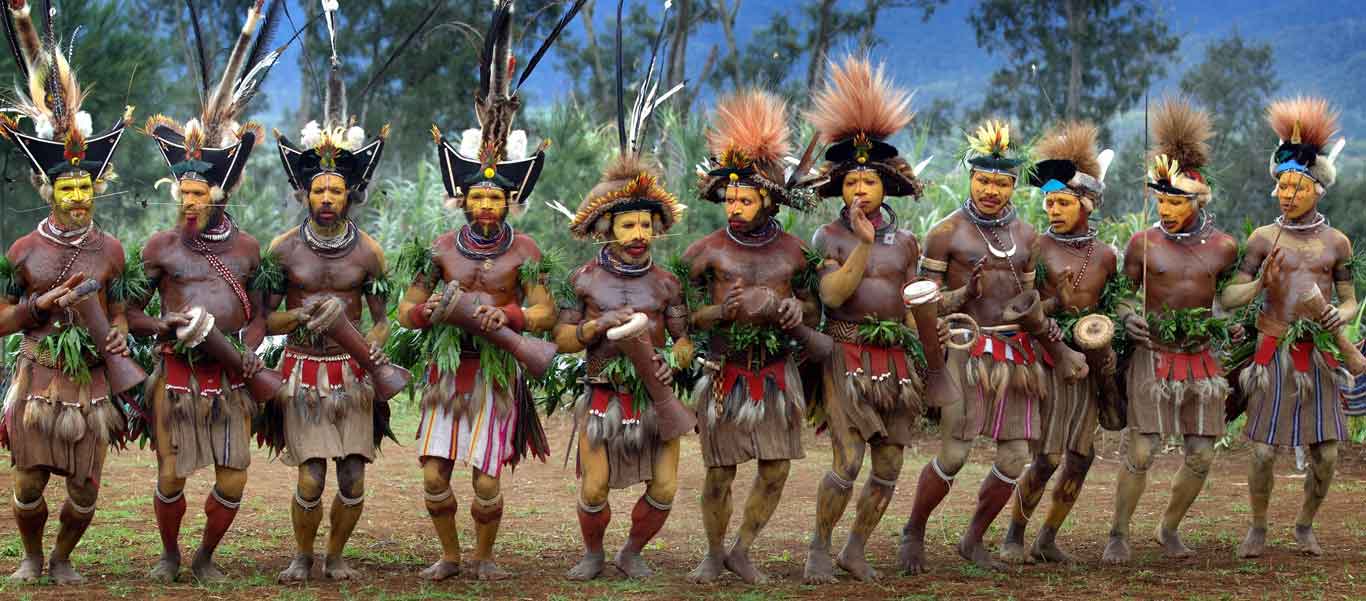In the image, taken outdoors, a group of eleven or twelve men stands shoulder to shoulder on a dirt and grassy area, with a lush forest and blue sky in the background. They appear to be participating in a tribal dance or ritual, as they hold Congo drums and have their faces painted a light yellow color. The men wear ornately decorated hats; some resemble pointy Napoleon hats adorned with peacock feathers, while others have blue bands and resemble pirate hats with pampas grass, in various shades from light to dark brown. Their attire includes skirts with red stripes, and their legs are adorned with strings just below the knees, mimicking the appearance of knee-high socks. Overall, their attire, painted faces, and synchronized stance contribute to the ceremonial atmosphere captured in this photograph.